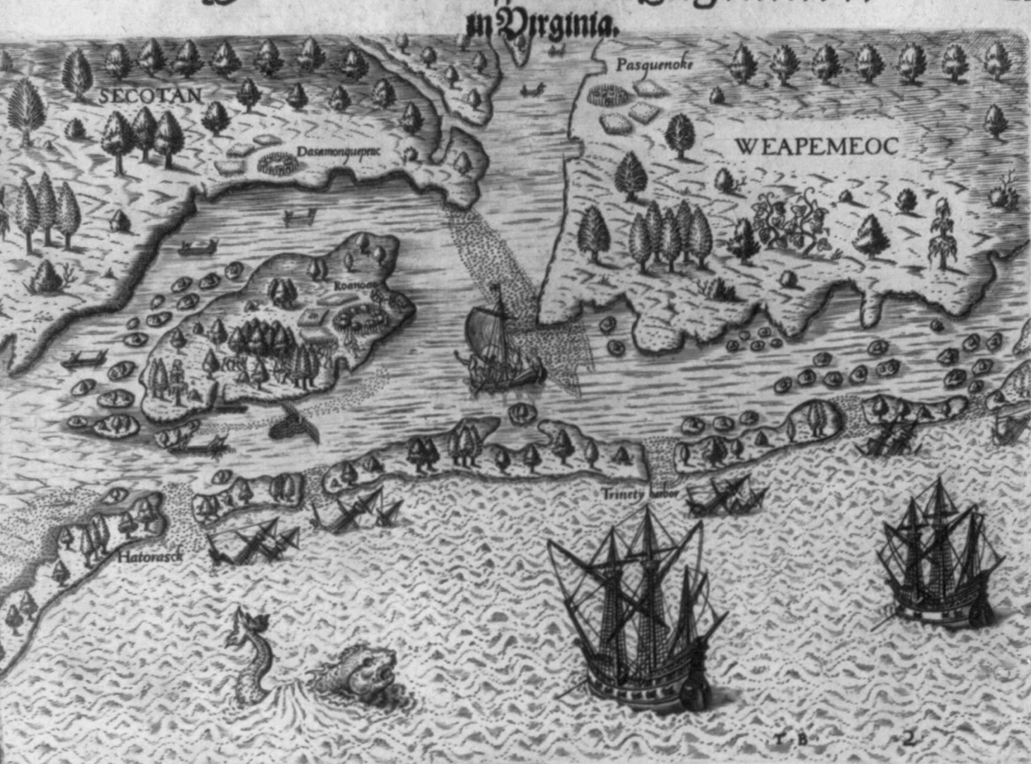The image features an intricately hand-drawn, ancient-looking black and white map, penciled in shades of gray. Dominating the lower section is a wavy body of water filled with detailed sailing ships, identifiable by their rigging but missing the sails. Towards the lower left, a menacing sea creature with a fish-like head and sharp tail emerges from the waves, next to several partially sunken ships, hinting at a shipwreck location.

Protruding from the water are raw, jagged rocks, contributing to the treacherous marine atmosphere. Moving upward, the water curves gradually to the middle right, ultimately leading to a broader expanse bordered by landmasses adorned with clusters of trees.

On the middle left, an island is positioned, encircled by a river branching out to meet the larger body of water. Encroaching into this waterway, a chain of smaller islands forms a natural barrier to the mainland, which has densely wooded regions.

Key locations are annotated: "M. Virginia" prominently tops the map, though only partially discernible. Additional placenames like "Weepi Myiak" (or possibly "Wepamiok") in the upper right-hand corner and "Secotan" in the upper left are visible. Another name, "Paskimoki," is marked near the center top, albeit harder to decipher clearly.

Overall, this captivating map merges art and cartography, offering a window into a possibly fictional or historical landscape rich with exploration details.